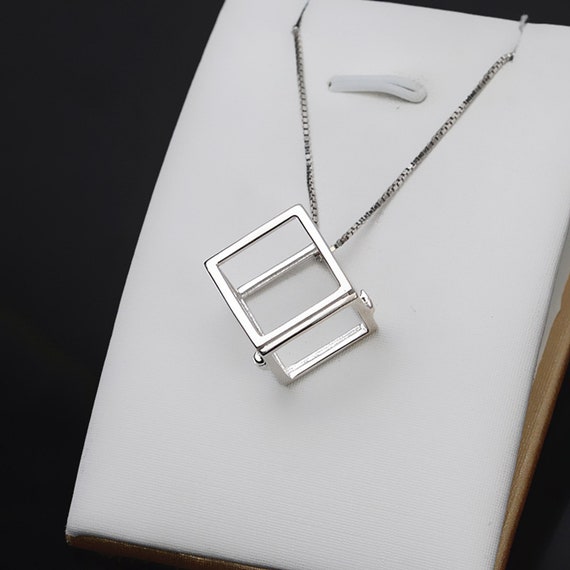The image displays a sleek necklace showcased on a white, cushioned triangular display set against a solid black background, reminiscent of a jewelry store setup. The necklace features a thin silver chain with a prominent, 3D silver square charm at its end. This charm has clear panels, revealing its inner space, suggesting it might be functional like a small box with hinges, possibly able to open. The display also includes a distinctive small white tab at the top for securing or hanging the necklace.